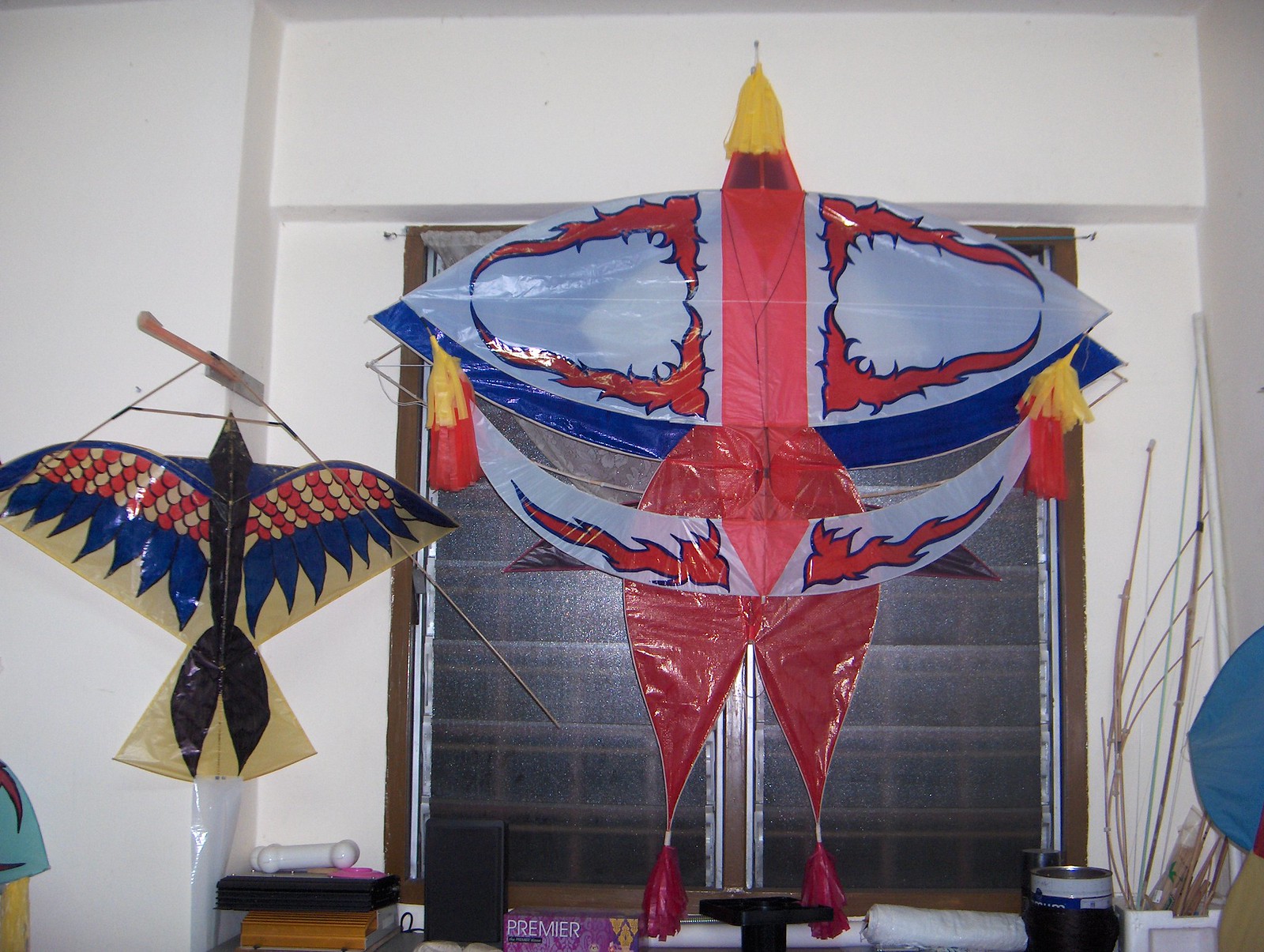In this detailed image, we observe two intricately designed bird-themed kites displayed indoors against a backdrop of frosted glass Jalousie windows. The kite on the right is the larger of the two, showcasing an oval-shaped design with a red rocket pattern running through its center, culminating in a white or yellow tip. This kite also features two red, upside-down triangular flaps adorned with red tassels. The smaller kite on the left resembles an eagle in mid-flight, its body predominantly black with striking feathered wings in red, white, and blue. Below the kites, there's a collection of miscellaneous items and empty containers scattered across a countertop or storage area, further emphasizing the room's eclectic decor.